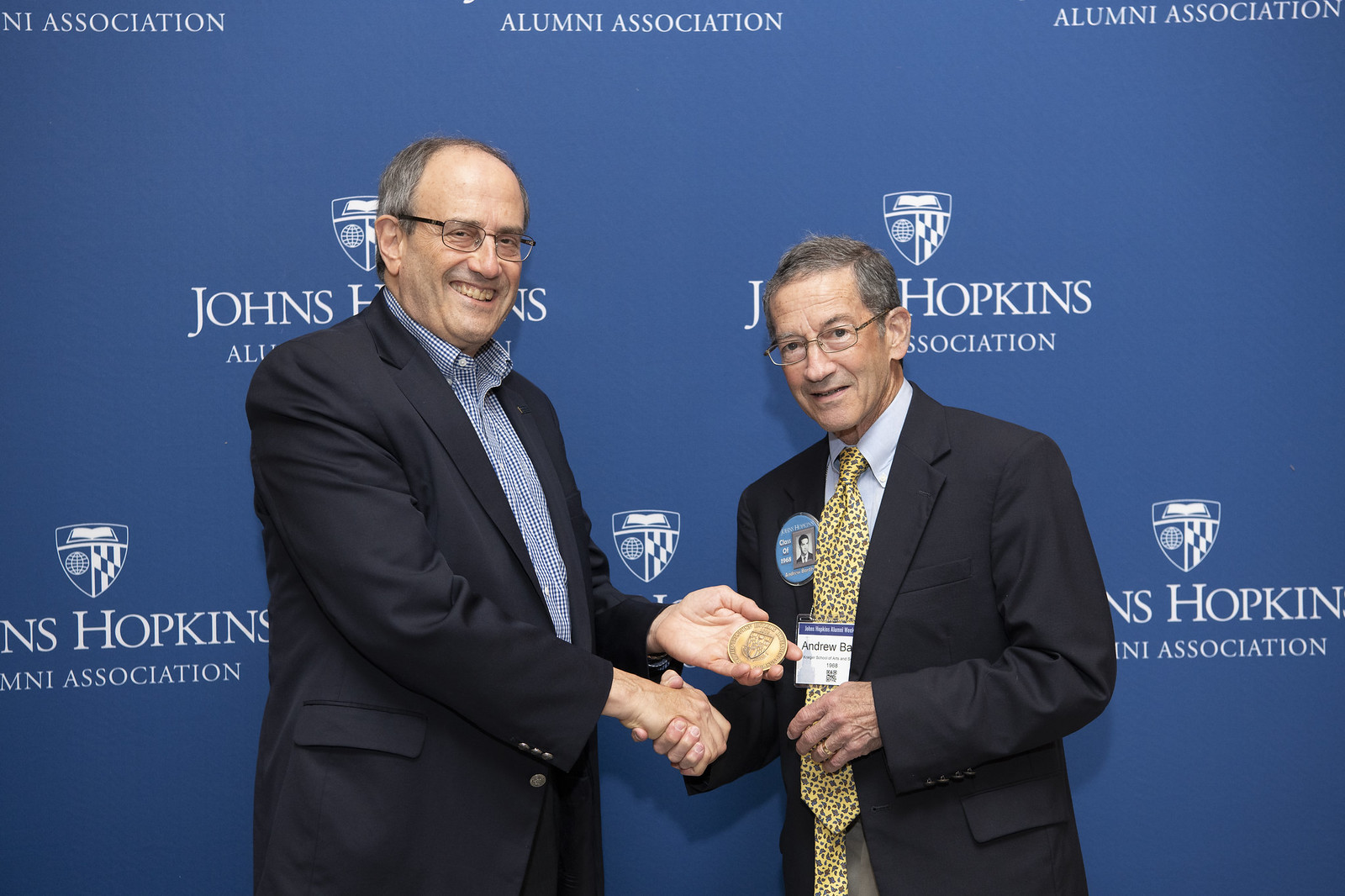In this color photograph, set indoors at an award ceremony, two middle-aged Caucasian men are captured shaking hands in front of a dark blue backdrop adorned with the repeated logo of the Johns Hopkins Alumni Association. The logo features white text and a shield containing an open white book, a globe, and a checker pattern in its segments. The man on the left, who is taller, balding, and wearing glasses, is dressed in a black business jacket over a blue and white checkered button-up shirt without a tie. He smiles at the camera while extending a large gold medallion towards the shorter man on the right. This shorter man is dressed in a black suit with a blue button-up shirt and a yellow leopard print tie, which is noticeably poorly tied. He also has a large blue button with a black and white photograph of a man on his lapel. Both men are exchanging a handshake with their right hands as part of the award presentation.